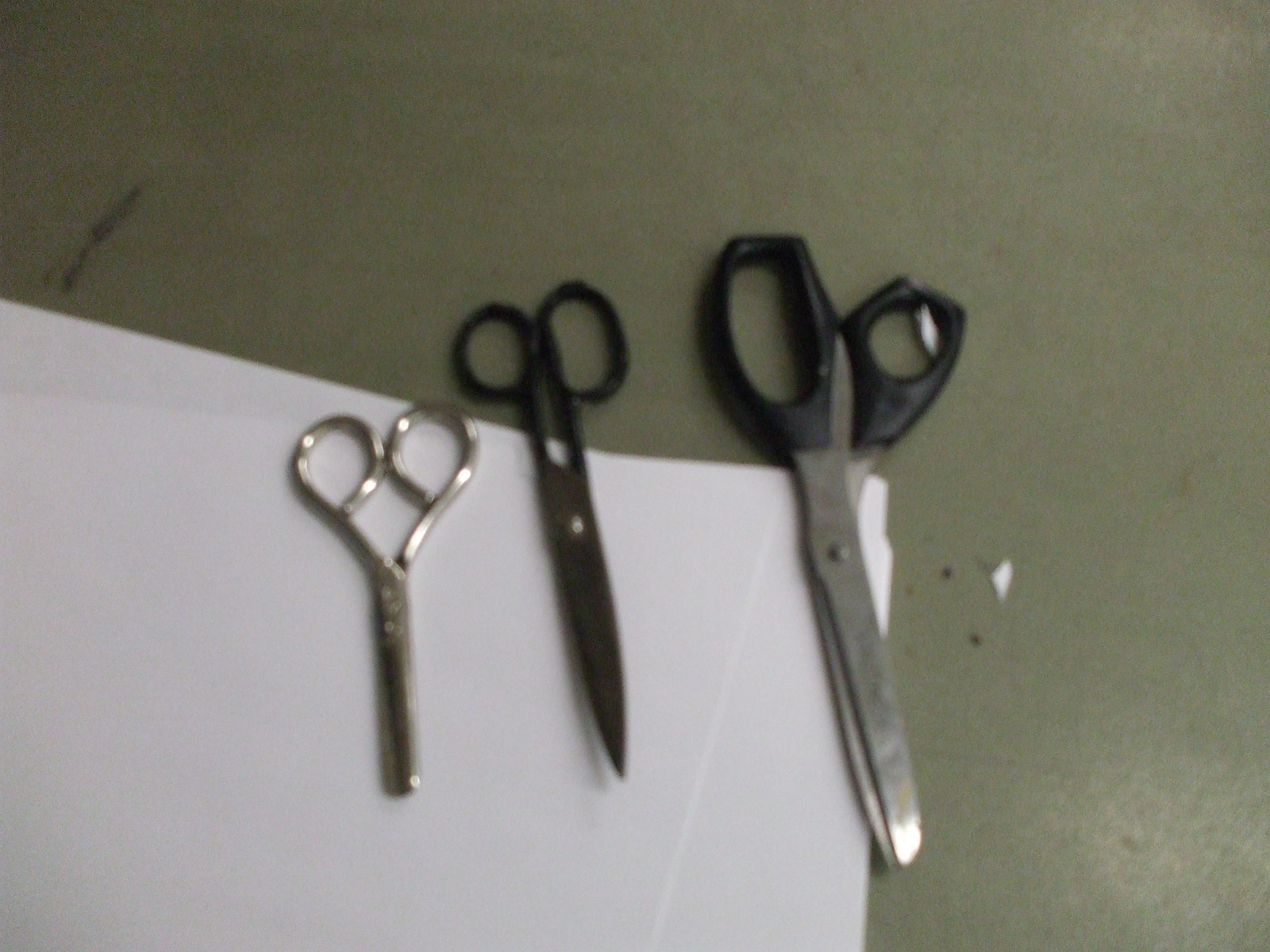This slightly out-of-focus photograph depicts three pairs of scissors resting on a gray surface, resembling a plastic tabletop commonly found in science classrooms. A stack of about four or five plain white sheets of paper partially covers the bottom left-hand corner of the image, elevating the scissors slightly, with some small paper scraps nearby. The smallest pair of scissors is all metal, silvery, with a rounded tip, suggestive of safety scissors often seen in children's classrooms. The middle pair, of medium size, features silver metallic blades with black-painted handles and ends with a pointed tip. The largest pair on the right has black plastic handles, though they appear misshapen, and long silver blades, also ending in a pointed tip. The photograph is dimly lit and slightly blurry, contributing to a somewhat unclear focus.